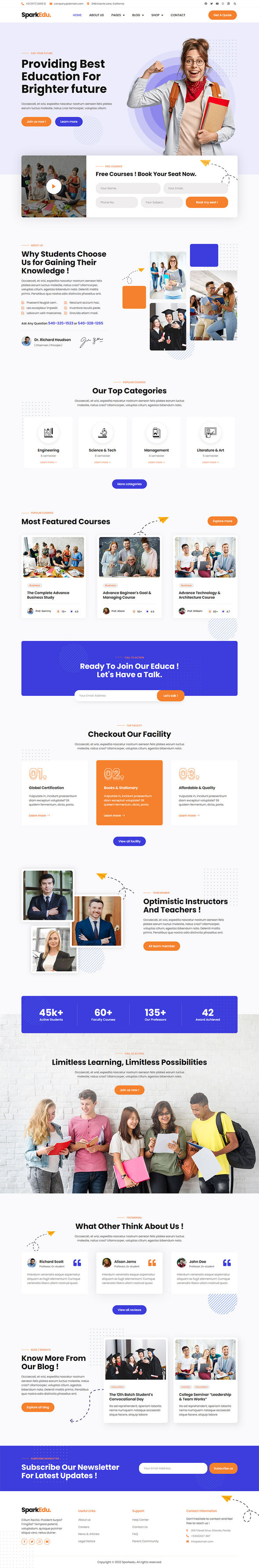The image depicts a lengthy and pixelated web page that is quite blurry. At the top of the page, there is some black text that is illegible, accompanied by the readable phrase, "Providing best education for brighter future." Below this, there are two buttons: one blue and one yellow. Prominently featured on the page is an image of an individual, possibly a woman or child, holding a stack of books and striking a strongman pose. The page also includes a clickable video link. The overall color scheme of the web page incorporates a lot of orange and blue tones. Additional photographs of children are scattered throughout the page. Towards the bottom, there is an orange box and another blue button, along with blue banners. One of the images near the bottom features high school students standing against a wall. Among them, one student is wearing a yellow outfit, another in green, one in pink, and one in white. Another student, who is blonde, is dressed in a jean jacket, white shirt, and gray pants.